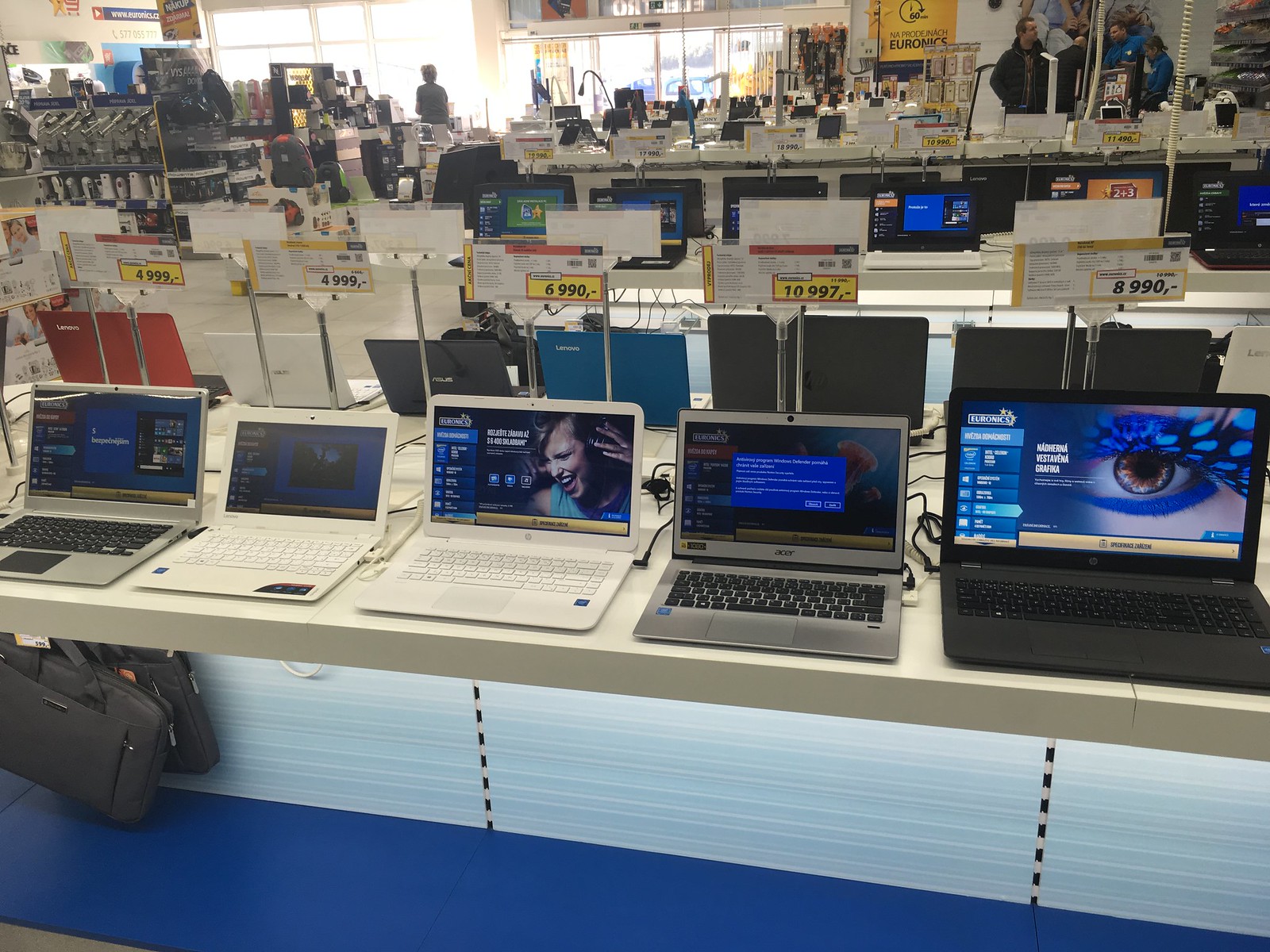This image, a color photograph, captures the bustling interior of an international electronics store. The store is well-lit, with light streaming in from the front doors, which are visible in the background. At the forefront, multiple rows of laptops of varying sizes and colors, including black, silver, white, and blue, are set up on several desks, each marked with price tags. The laptops are displayed open, with screens turned on, and underneath them are some bags. Adjacent shelves along the store's walkway hold additional items, such as keyboards and laptop cases displayed on the left side.

In the background, a service desk staffed by employees interacting with customers can be seen. Further back, several posters with non-U.S. text, like "Na Praninach Uranix," adorn the walls, hinting that the store is located outside the U.S. The spacious store is busy with a few customers shopping and engaging with employees, reinforcing the active, customer-centric atmosphere.